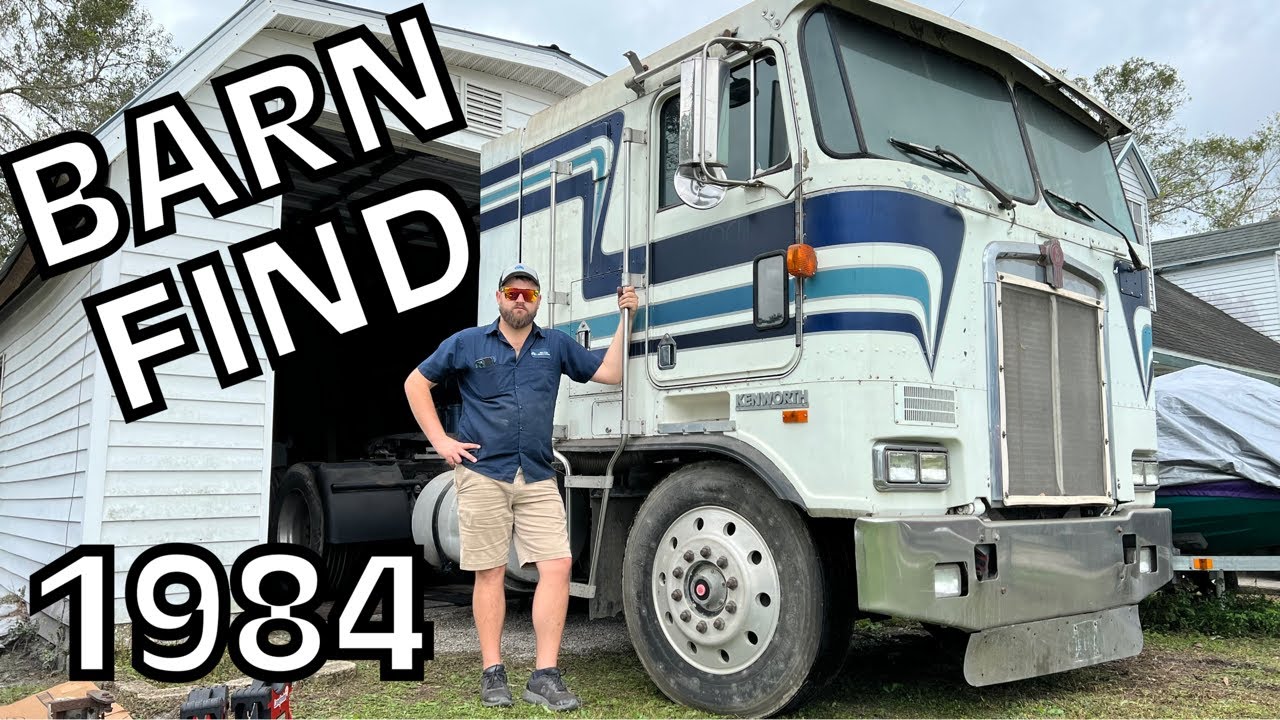A thumbnail-style photograph depicts a Caucasian man standing outside next to a semi-truck partially pulled out of a large, white, barn-style garage. The man, wearing a dark blue cap, reddish-brown sunglasses, a dark blue short-sleeve shirt with a white logo over the left breast, tan shorts, and black sneakers, is positioned to the left of the truck. He stands with his right hand on his hip while holding the passenger door handle with his left hand, which is above his head. The semi-truck, an older 18-wheeler from the 1980s, features dark and light blue pinstriped detailing running from the front, below the driver's window, and extending over the rear of the cab. The text "Barn Find" appears prominently in white with a black outline on a diagonal across the man's left side, accompanied by "1984" placed more subtly in the bottom left corner of the image. The truck is so large that its front extends near the bottom right corner of the photograph, while the rear remains inside the garage. There also appears to be a covered boat behind the truck, further enhancing the scene of a significant vintage discovery.